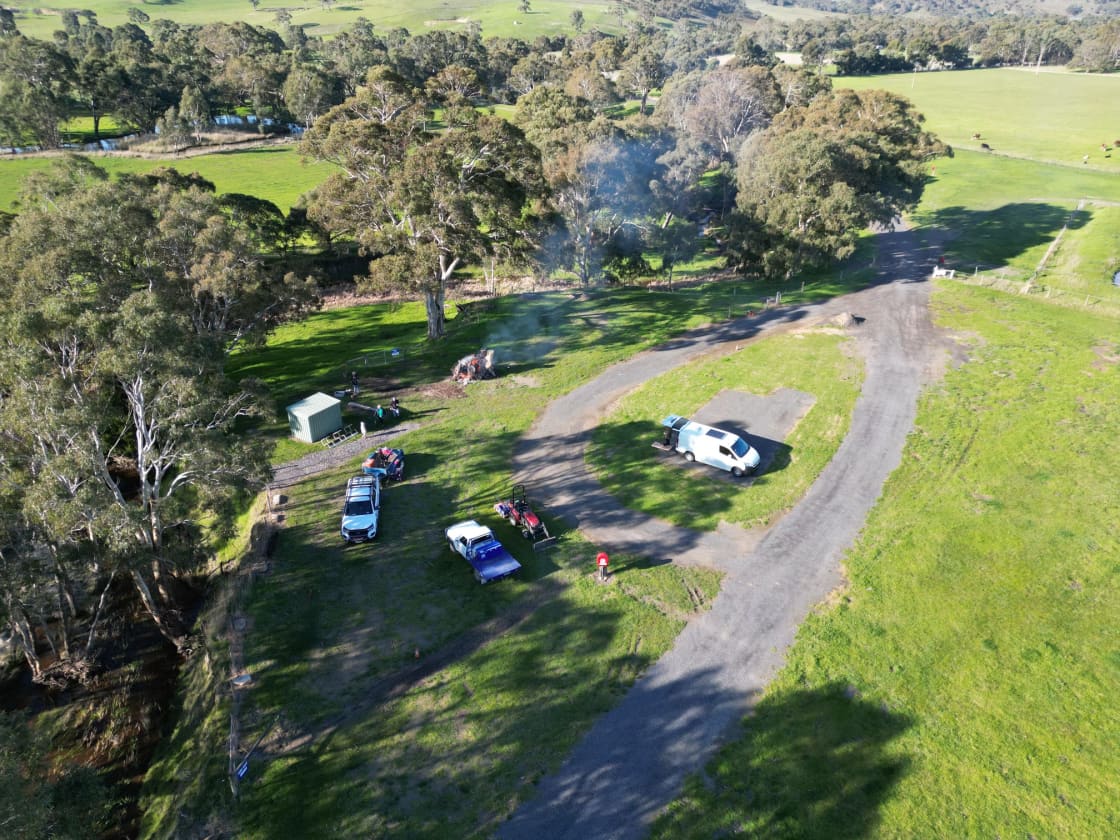This aerial photograph captures a lush, verdant park-like property characterized by expansive green grass and large, old-growth evergreen trees. The landscape is punctuated by a looping pavement path that forms a '9' shape in the center of the field. Three vehicles are parked within this loop: a white van with its trunk open, a white vehicle near some tents, and a smaller white and blue vehicle, possibly indicating a camping setup. Additionally, a red tractor is visible, hinting at agricultural activity or maintenance. A smoke trail ascends into the sky, suggesting an ongoing barbecue or cookout. In the backdrop, a serene lake or river meanders along the edge of the property, with rolling hills and more trees defining the distant horizon. Cows can be seen grazing in a far section of the field, adding to the rural, bucolic charm. Scattered small fences line parts of the road, encapsulating a picturesque and seemingly serene day.